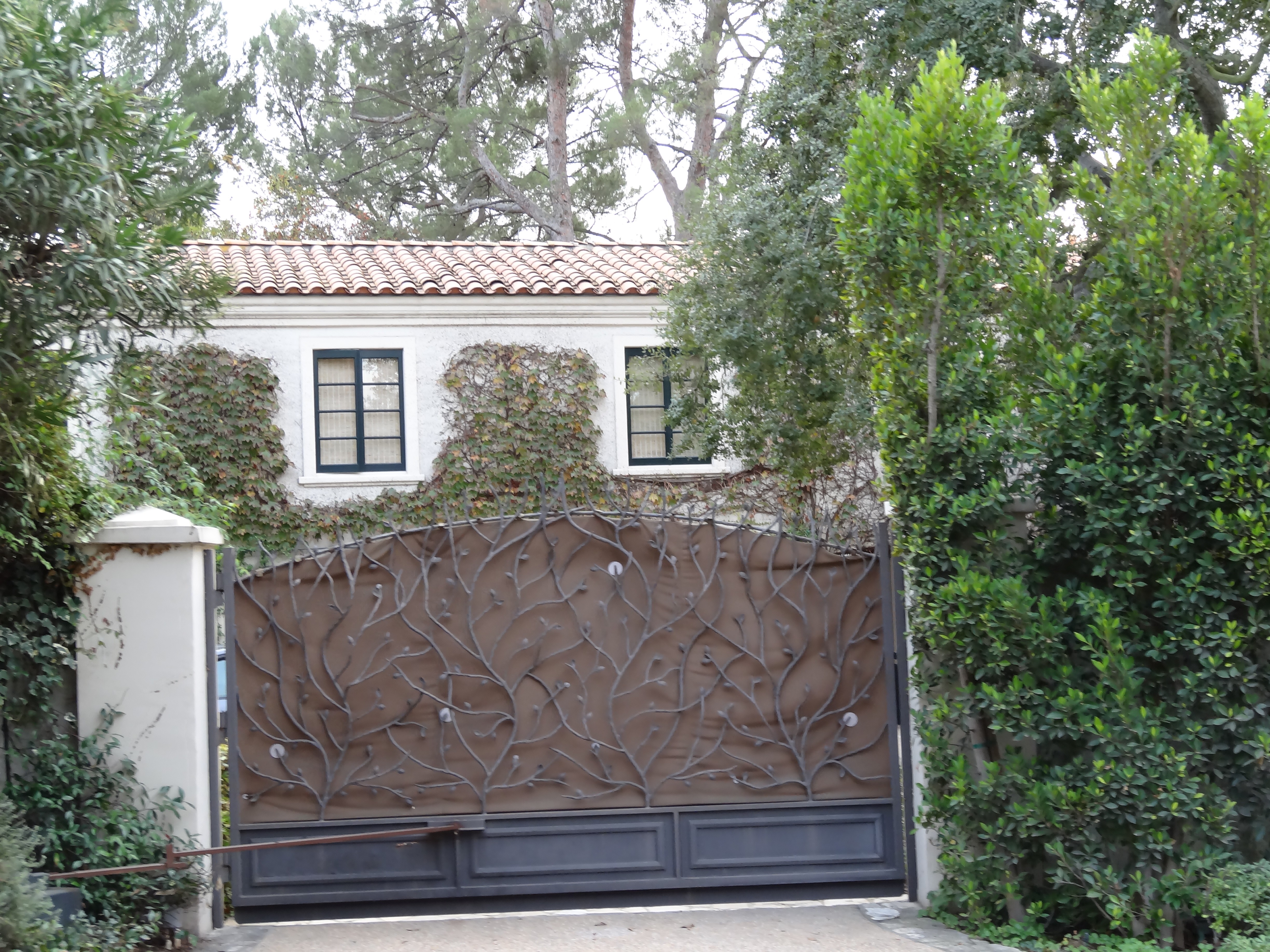The photograph depicts a white house with a red shingled roof, partly obscured by a central gate. The gate, adorned with vine-like decorations in black steel and featuring a solid brown cover at the top, draws the viewer's focus. Flanking the gate are beige columns that match the house's exterior. Ivy, both green and brown, climbs up the facade of the house, hinting at both life and decay. The house features two black window panes with beige interiors. Surrounding the scene are lush green trees and bushes, adding a vibrant natural frame to the setting. The overall composition, captured in daylight, emphasizes the gate as the focal point, with the house and greenery providing a rich, detailed backdrop.